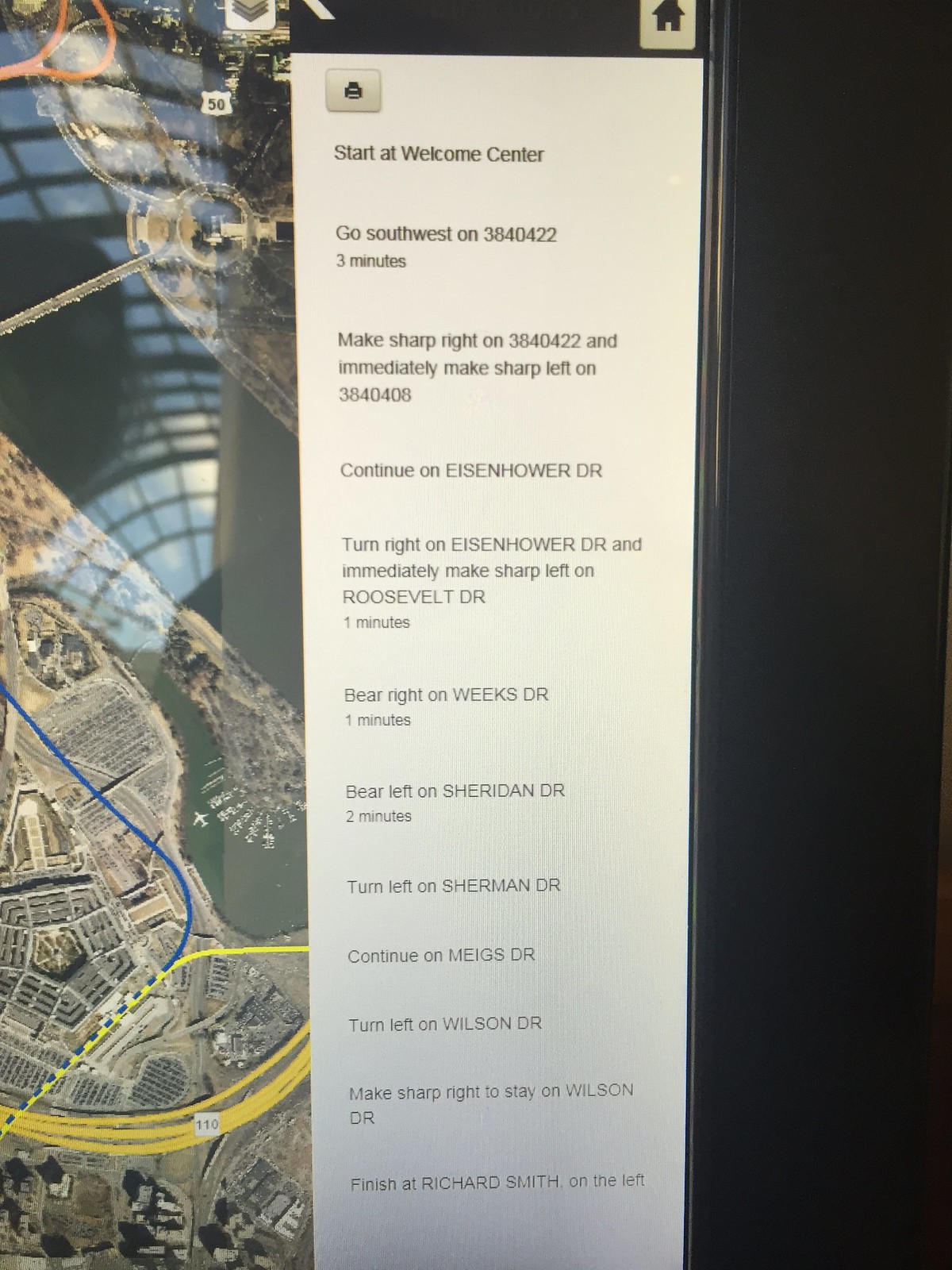This photograph captures a digital kiosk or desktop computer screen, primarily displaying a detailed directional guide. The screen robustly features a long column of printed directions in black text on a white background, starting from the Welcome Center and concluding at Richard Smith. Adjacent to these written directions, the screen exhibits an aerial, satellite-like map view of a city landscape, including roads, airports, bridges, and a river, with highlighted routes in yellow and blue lines. The print button, prominently situated at the top of the directional field, highlights its functional purpose. Reflected on the glass screen is a partly cloudy blue sky, hinting at an arched, dome-like glass structure commonly found in public spaces such as hotels or shopping malls. This intricate kiosk setup, likely positioned in a public area, serves as a navigational tool for its users.